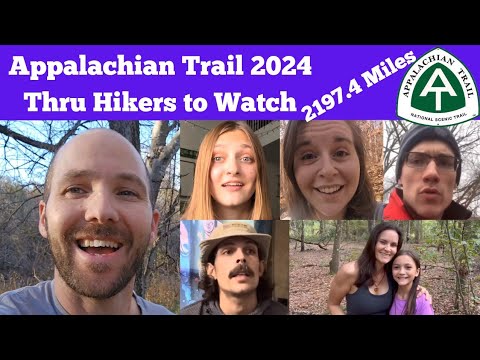The photograph features a collage of individual portraits against a black background, resembling a presentation slide. At the top, a purple banner with white letters reads, "Appalachian Trail 2024 THRU Hikers to Watch - 2197.4 miles." The banner is accompanied by an Appalachian Trail patch featuring a green triangle with a tree outline and the text "National Scenic Trail."

The collage includes six photographs of hikers, each depicted in a well-lit, smiling portrait. Starting from the left, the largest image shows a bald man with a beard, dressed in a gray shirt, standing beside a tree. Next to him, in the top row, is a warmly lit portrait of a blonde woman, likely in her 30s. Beside her is another smiling woman, also in her 30s, appearing to be outdoors. Continuing to the right is a man with glasses and a hat.

In the lower row, from left to right, there is a mother-daughter duo embraced in a hug; the mother is in her 30s, and the daughter appears to be around nine or ten years old. Completing the collage is a man with a mustache, wearing a hat, posing in an outdoor setting. Each hiker's photograph is carefully placed to highlight their joyful expressions and convey the spirit of adventure on the Appalachian Trail.